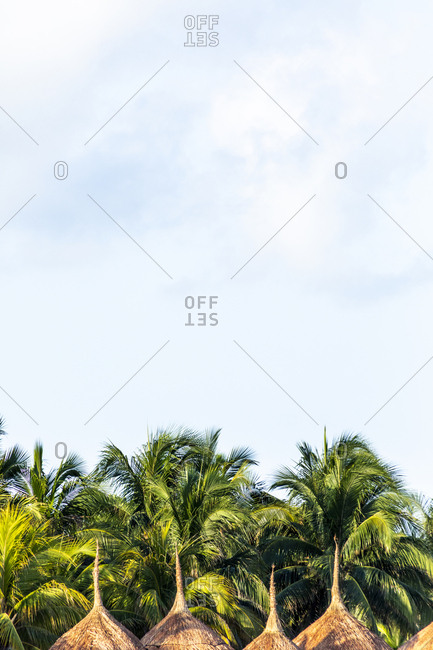The image features a rectangular composition dominated primarily by a light blue sky, tinged with turquoise hues and scattered with wispy white clouds. The upper portion of the image contains the word "offsets" repeated with long dashed lines leading to the digit zero, creating a triangular pattern. These elements are outlined in gray and stamped across the entire sky, giving it a distinctive watermark-like appearance. Below the sky, the lower portion of the image is filled with a lush cluster of palm trees, showcasing long fronds in a vibrant green. The trunks of the palm trees are visible, marked by their brown branches. In front of the palm trees, there are several huts with pointy tops, appearing to be constructed from natural materials, possibly hay or dirt, and tinged in brown. The overall scene is a harmonious blend of natural elements and graphic overlays.